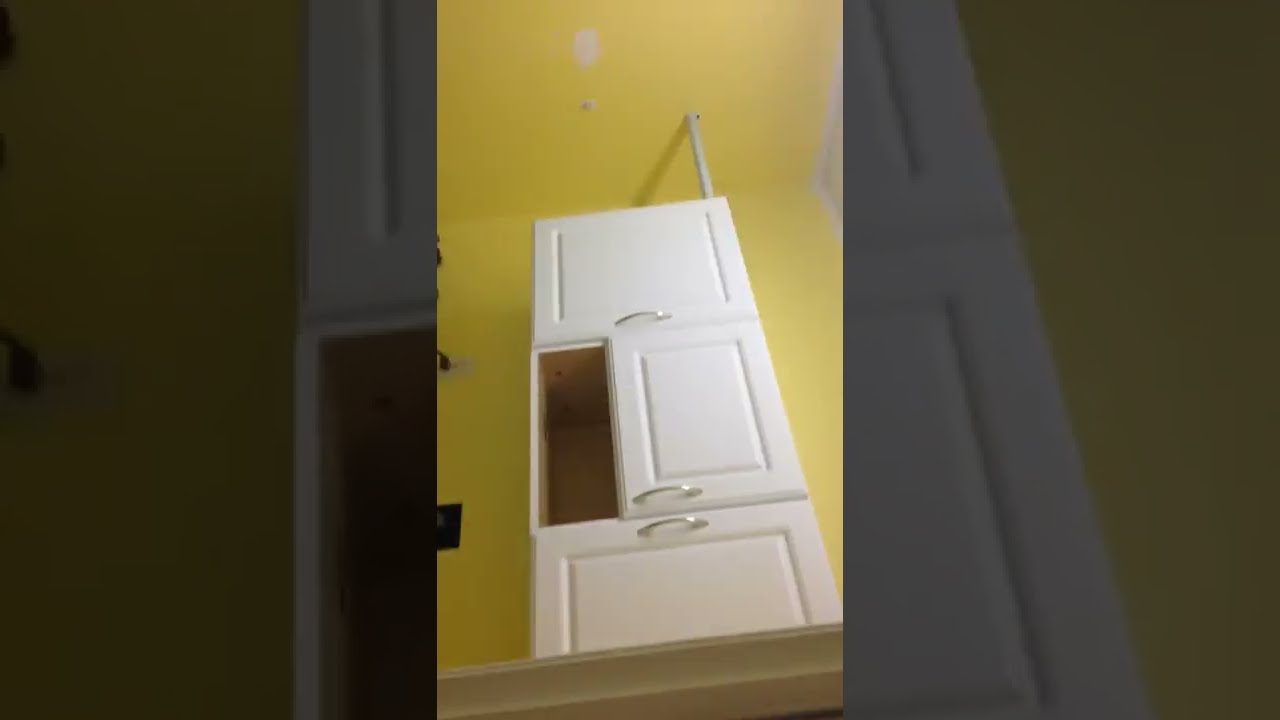This image captures an indoor scene with a bright yellow wall and ceiling. Central to the photograph is a series of white cabinets stacked on top of each other. Each cabinet has distinct features and forms a cohesive arrangement. The handles on these cabinets are silver and rounded in shape. The top and bottom doors are square, both with silver handles; the top door has its handle positioned at the bottom, while the bottom door’s handle is at the top. The middle section is divided into two parts: on the right, there is a white cabinet door similar to the top and bottom ones, with a silver handle off to the right hand side; on the left of this middle section, there's an open shelf revealing bare wood. Additionally, a silver metal bar is seen extending from the top right of the cabinets up to the ceiling, possibly providing support. The overall composition is neat and minimalistic, focusing on the contrast between the vibrant yellow walls and the clean white cabinetry.